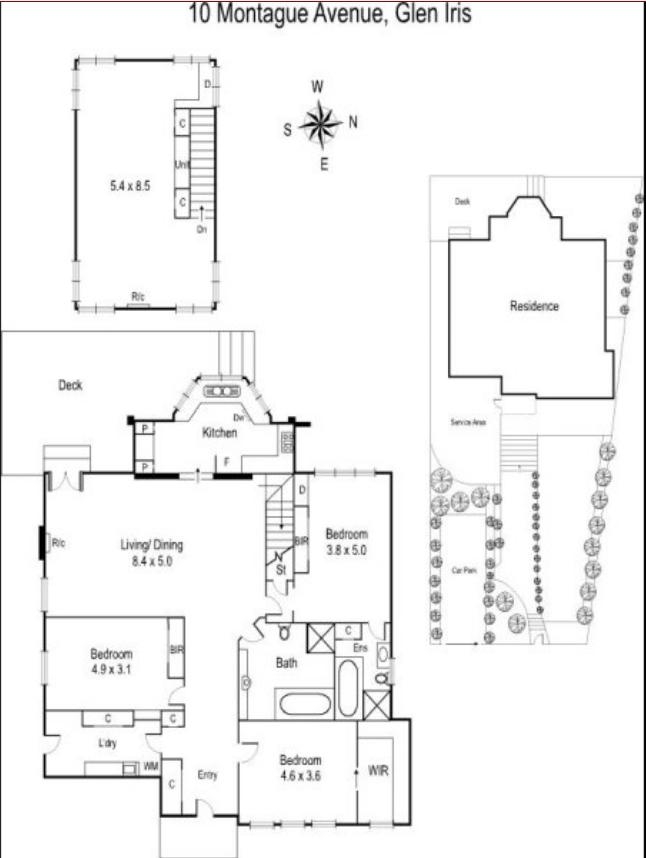This detailed floor layout plan is for a property located at 10 Montague Avenue, Glen Iris. The plan utilizes a compass indicating the cardinal directions (north, south, east, west) for orientation. The building is divided into three distinct sections.

The top section features a small rectangular structure measuring 5.4 meters by 8.5 meters. Moving downwards, the main building of the property comes into view. 

Upon entering the main building, there is an entryway. To the left of the entry, a laundry room can be found. On the right side, there is a bedroom equipped with a walk-in closet. Continuing down the hallway, a smaller bedroom with a modest closet is located on the left. Across from this room, on the right, is a bathroom featuring a bathtub.

Advancing further into the house, an expansive living and dining area unfolds, with dimensions of 8.4 meters by 5 meters. The kitchen is situated further into the house, occupying its own enclosed space. 

Adjacent to the dining area on the right, there is the master bedroom, which includes an ensuite bathroom. 

There are stairs accessible from the main building, presumably leading to the first section, which could be an upper floor or a rooftop area. 

On the right side of the layout, the overall design of the entire property is visible, providing a comprehensive view of the building's layout.